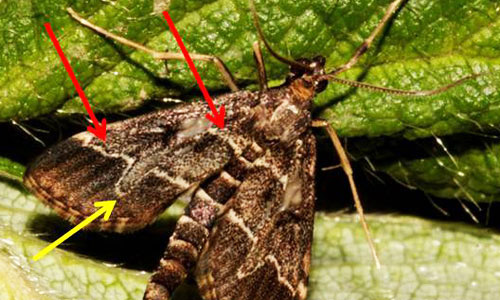This image depicts a close-up view of a brown moth resting on green leaves, possibly taken outdoors or under a microscope for enhanced visibility. The moth features a pattern of white stripes along its brown body, accentuated by its prominent antennas and long legs. The photograph includes two red arrows pointing to different sections of the moth's body from above, highlighting specific parts of the color scheme, while a yellow arrow on the lower left points upwards towards a particular design on the moth's wings. The moth's body also exhibits some white hairs, adding texture to its overall appearance.